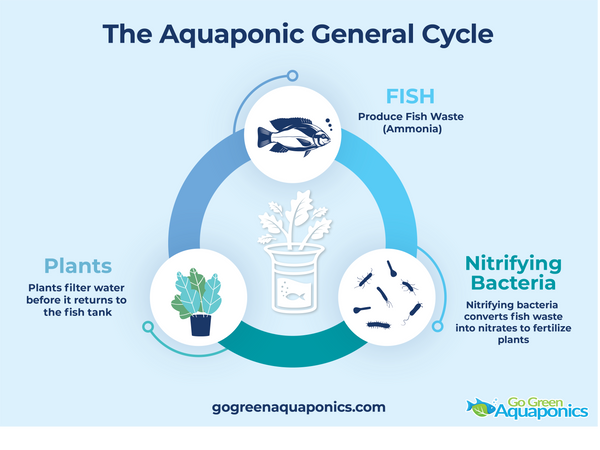The image is a color illustration from the website GoGreenAquaponics.com, prominently displaying "The Aquaponic General Cycle" title in large, bold blue font. The background is a pale aqua, complementing the schematic's circular diagram, which is outlined in various shades of blue: cornflower blue, turquoise, and teal. At the bottom and in the bottom right corner, the logo and website of Go Green Aquaponics are visible, with the company name in green and turquoise and a logo featuring a turquoise fish overlaid with a green leaf.

The schematic consists of three key components arranged in a triangular layout within the circle. At the top, a blue cichlid fish is depicted inside a white circle, labeled "Fish," with the annotation "produce fish waste (ammonia)." Moving clockwise, the next white circle contains blue illustrations of nitrifying bacteria, labeled "Nitrifying Bacteria," with the explanation "nitrifying bacteria convert fish waste into nitrates to fertilize plants." The third white circle shows plants with oak leaf-shaped leaves growing in a blue pot, labeled "Plants," and notes that "plants filter water before it returns to the fish tank." 

At the center of the schematic, a white outline drawing of a cylindrical tank with fish and plants emphasizes the continuous cycle of water and nutrients. The overall design effectively illustrates the aquaponic cycle, reinforcing the sustainable interaction between fish, bacteria, and plants.